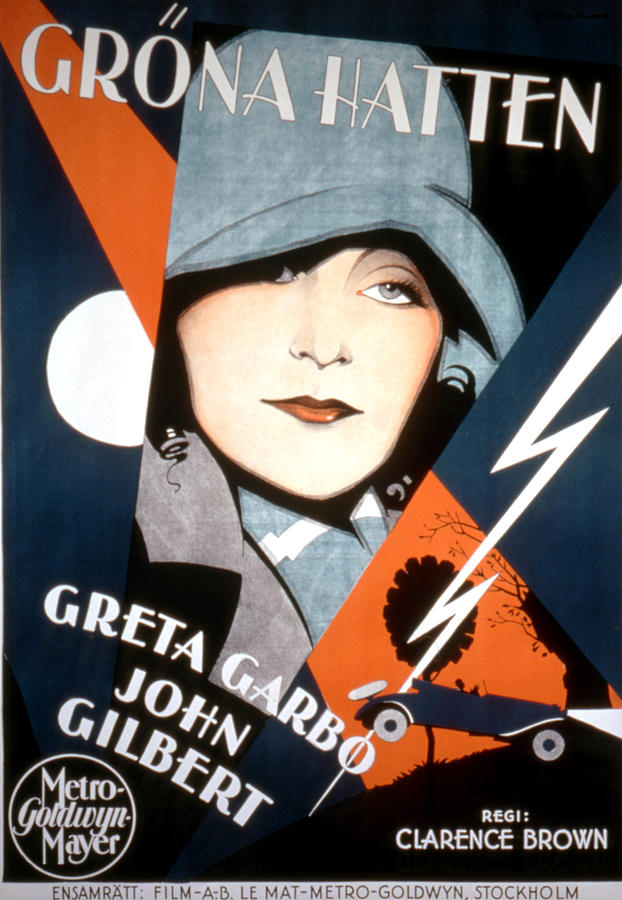The image is an advertisement for a movie, presented in portrait mode. It appears to be a vintage poster from the 1940s or 1950s, in full color, and not in English. Dominating the composition is the portrait of a mysterious light-skinned woman, possibly dressed in period attire from the 1940s. She wears a dark gray bucket-style hat that covers her right eye, a blue and white scarf, and red lipstick. Her enigmatic expression is set against a dramatic background: a lightning bolt shoots through the right side of the image and a bright red stripe diagonally cuts from the top left-hand corner into her face. The backdrop also includes a moon and a vintage car, likely from the 50s. Key names are prominently displayed: "Greta Garbo" and "John Gilbert" in the top left corner, and "REGI: Clarence Brown" in the lower right corner. The Metro-Goldwyn-Mayer logo appears as a circle in the upper left, and in a gray strip at the bottom, a text likely reads "ENSAMRATT: FILM / A / B LE MAT / Metro Golden Stockholm," indicating the studio or distributor.